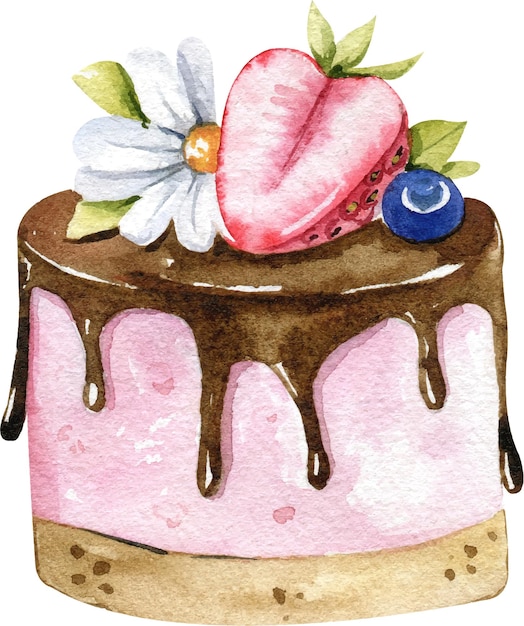This illustration, reminiscent of watercolor technique, features a pink, cylinder-shaped dessert cake with a light brown crust at the base, covered in chocolate frosting that drips down all sides. Atop the cake are intricate details: a half-cut strawberry with visible seeds and three green leaves, accompanied by a small, blue blueberry. Next to the strawberry is a delicate white flower with a yellow center and two green leaves. The chocolate frosting forms six distinctive drips, enhancing the vibrant yet faded, cartoony style of the painting, similar to clipart. The background is plain white, highlighting the dessert's subtle details and colors.